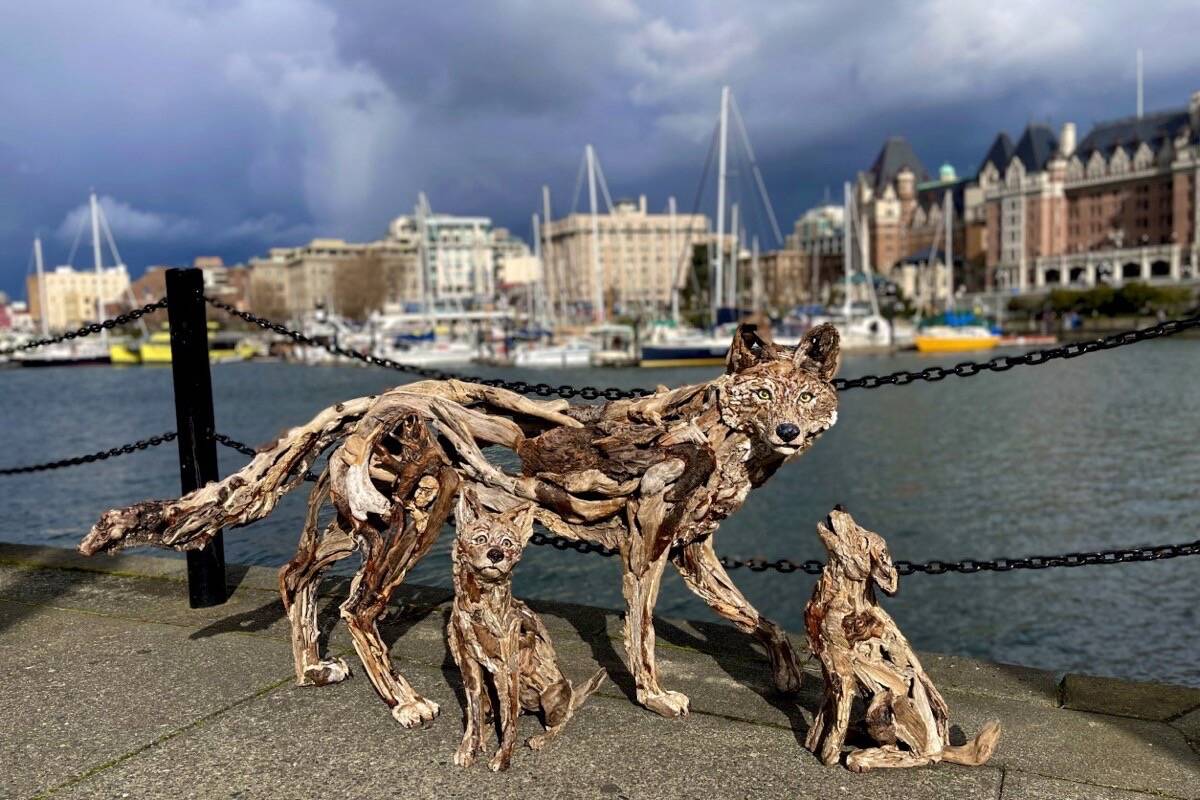This photograph captures a striking sculpture set against the backdrop of a serene bay or lake, with a cloudy sky, a skyline, and various boats slightly out of focus on the dark blue and grayish water. In the foreground, a black chain fence attached to a post emphasizes the outdoor setting. The sculpture features a lifelike depiction of a mother wolf and her two cubs, seemingly crafted from weathered, curved, and smooth driftwood, giving them an intriguing mix of transparency and decay, as if their fur and skin have eroded away to reveal their bones and faces. The mother wolf stands resolutely, gazing directly into the camera, while one cub sits at her side, calmly looking forward. The other cub appears frozen in mid-howl, head lifted towards the sky. The nuanced colors and textures of the driftwood add to the lifelike appearance, making it a compelling piece of art.